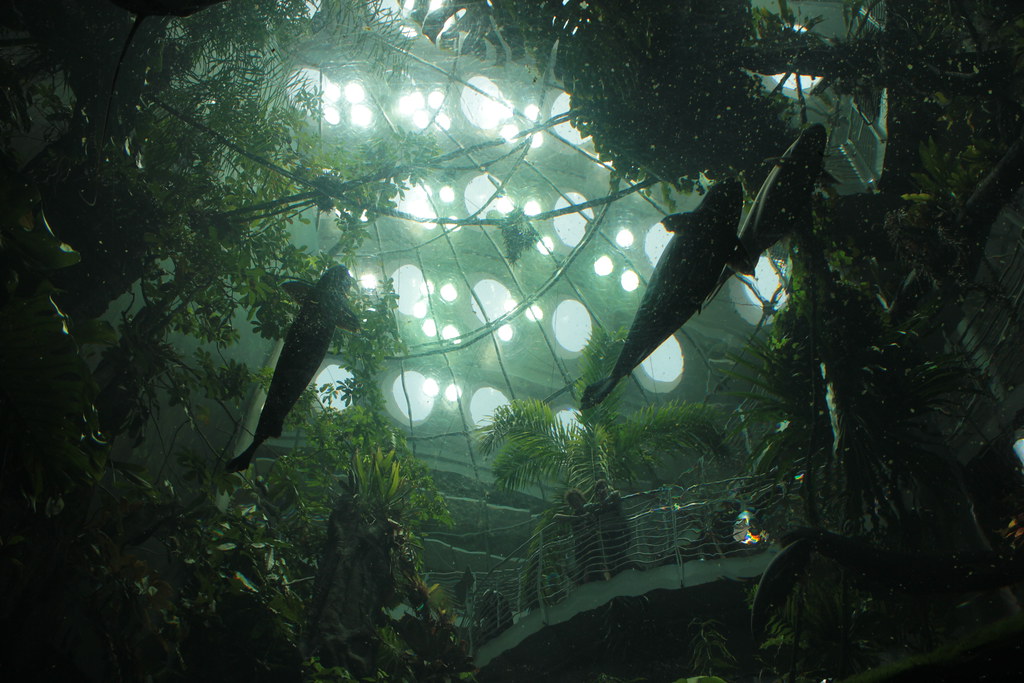The image depicts an underwater view inside a large aquarium exhibit, likely within a zoo or nature reserve. The photo captures the scene as if taken by a scuba diver, showcasing three large sea creatures—possibly whales or sharks—swimming gracefully above the camera. The water gives off a bluish-green hue, creating a serene and immersive atmosphere. Above the water, a transparent dome with circular skylights allows natural light to filter into the exhibit. Through the dome, spectators can be seen standing on a bridge-like structure, peering down at the aquatic scene below. The environment is surrounded by lush greenery, including numerous palm trees in the distance, enhancing the tropical and enclosed nature of the exhibit.